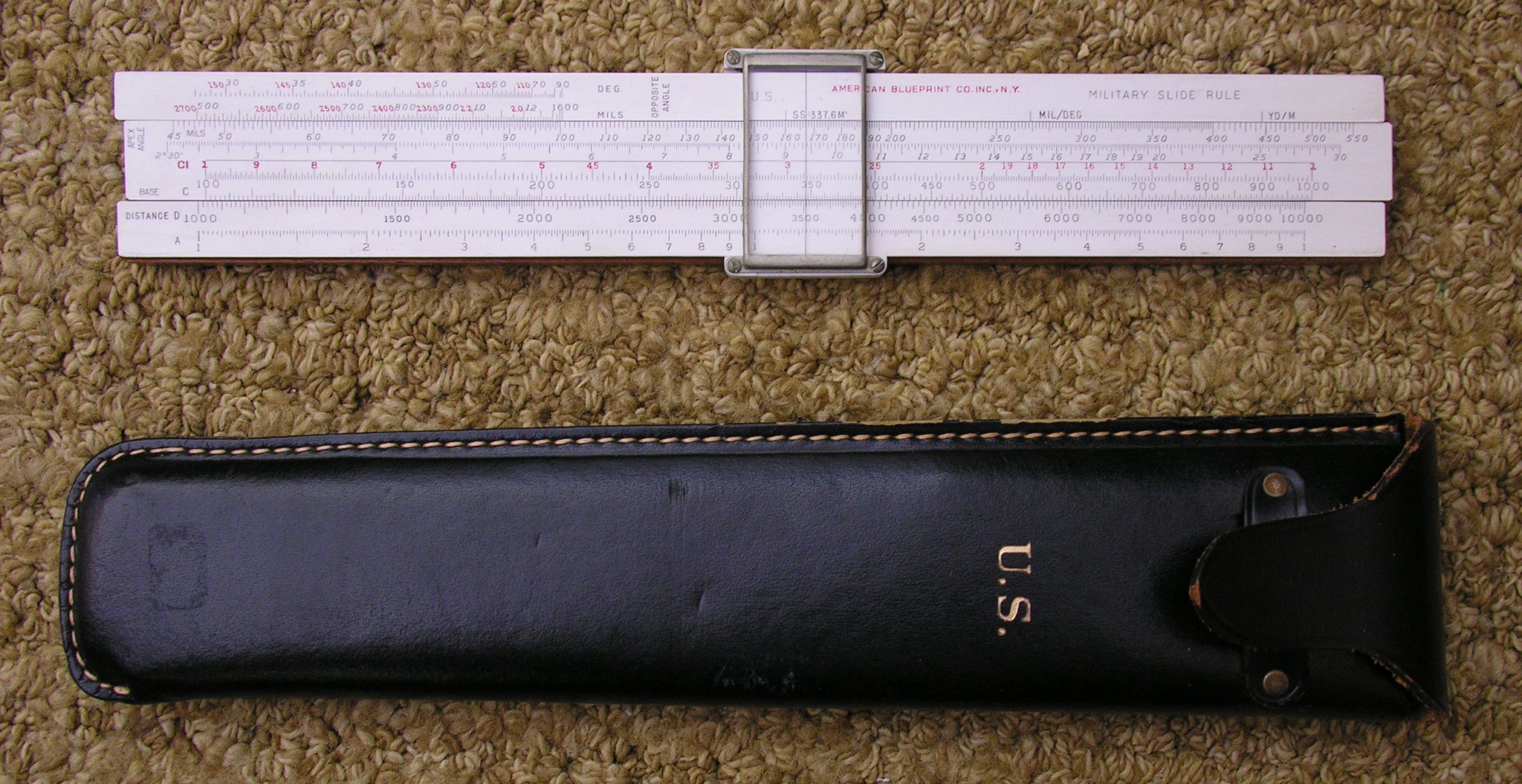The image is a narrow, horizontal rectangular photo featuring a classic slide rule and its accompanying leather case. The backdrop appears to be a fuzzy brown carpet. At the top of the image is a nearly closed slide rule, with its central sliding part edged in silver. The slide rule, marked with "American Blueprint Company" in red, has a clear sliding cursor for precise measurements. Below the slide rule lies a dark brown leather case, inscribed with gold letters that read "U.S." The case, likely designed to hold the slide rule, adds a touch of vintage craftsmanship to the scene. Both the slide rule and the case are positioned on their sides, emphasizing their complementary relationship.